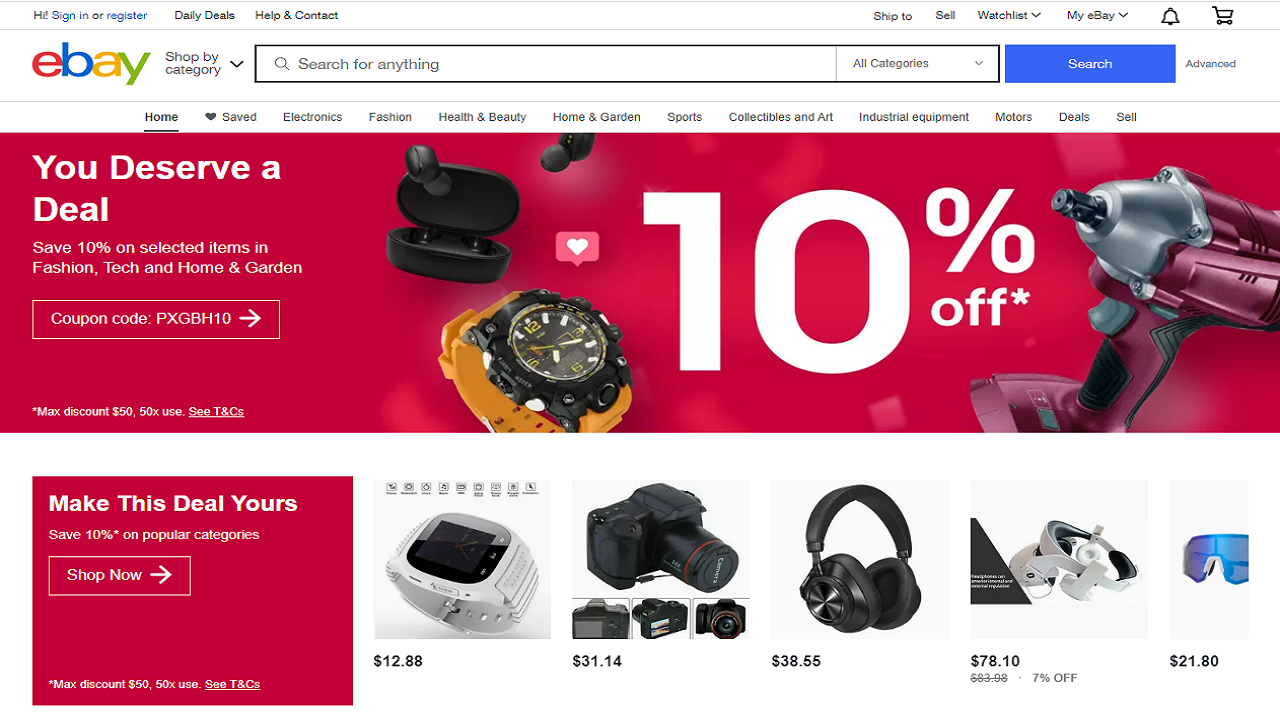This image showcases the eBay homepage. Prominently at the top, the iconic eBay logo is displayed with the letters 'e', 'b', 'a', and 'y' colored in red, blue, yellow, and green respectively. Just below the logo is a navigation bar, featuring options such as "Shop by category," a white search bar with the placeholder text "Search for anything," and a blue search button. Users can filter their searches by various categories.

The navigation tabs on the homepage include: 
- Home
- Saved (accompanied by a heart icon)
- Electronics
- Fashion
- Health & Beauty
- Home & Garden
- Sports
- Collectibles & Art
- Industrial Equipment
- Motors
- Deals
- Sell

Further down, a promotional banner with the message "You deserve a deal" is featured in white text against a background. This banner advertises a 10% discount on selected items in the Fashion, Tech, and Home & Garden categories with the offer of a coupon code, highlighted with a white arrow. An asterisk at the bottom indicates further details: "max discount $50, 50 times use, terms and conditions."

Highlighted below the banner are various items available for the 10% discount, including a power drill, a watch, and headphones, with the caption "Make this deal yours." The section encourages users to "Save 10% on popular categories" with a "Shop now" button visible. Some of the listed sale items include a camera priced at $31.14, headphones for $38.55, and a white headset for $78.10, among other products.

The homepage visibly lists a diverse range of items for sale, catering to different interests and needs.